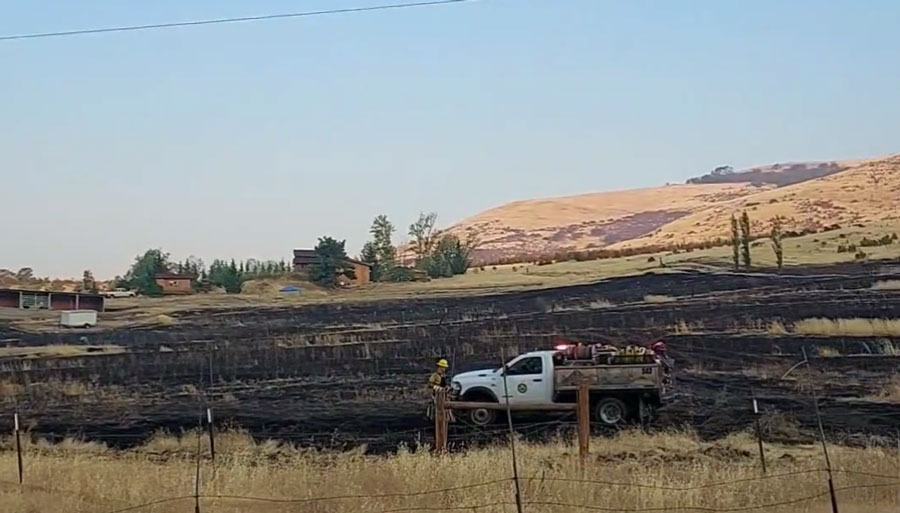The image features a clear, light blue sky with an electrical wire running from the upper left corner to the middle top. In the foreground, there is a white pickup truck with a brown flatbed and side barriers, loaded with construction materials. A man in a yellow hard hat stands in front of the truck, suggesting ongoing or impending construction work. The scene also includes a fence at the front with some green grasses behind it. The mid-ground showcases several mounds of dirt arranged in rows, and a couple of buildings, possibly houses or barns, to the left middle area. The background displays a mountainous terrain on the right side, characterized by yellowish grass, sparse patches of dirt, and few trees. To the left of the mountains, more trees are visible, which appear thin and sparse, adding a touch of wilderness to the scene.